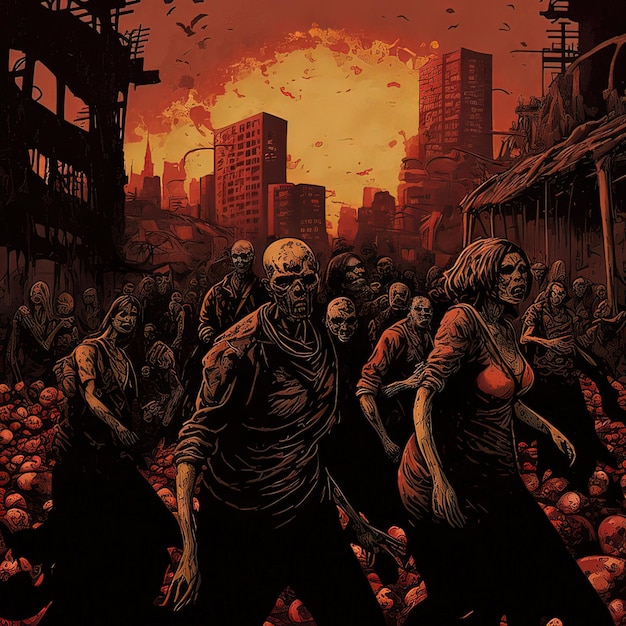This haunting image, seemingly a frame from an apocalyptic graphic novel, emanates a chilling, nightmarish aura rooted heavily in dark reds that saturate the scene. At its core lies a smoldering cityscape, where towering flames rise ominously into the air, casting a fiery glow over a backdrop of dilapidated skyscrapers and structures barely reminiscent of their former grandeur. The skyline is punctuated by the eerie, indistinct silhouettes of what might be birds, adding a foreboding touch against an infernal sky.

Dominating the foreground, skeletal figures with ghastly, skull-like faces manifest en masse, their bony, elongated limbs protruding from tattered, antique clothing. These ghoulish entities, evoking imagery of Night of the Living Dead, seem to teem from the depths of a world laid to waste, their numbers swelling into what could be hundreds, clustered and confined ominously to a flower bed that appears barren and desolate. The apocalyptic nature of the scenery is further emphasized by the sidewalk or street, strewn with what looks like rocks or perhaps skulls, enhancing the dystopian atmosphere as these undead specters appear to flee the inferno of their vanquished city.